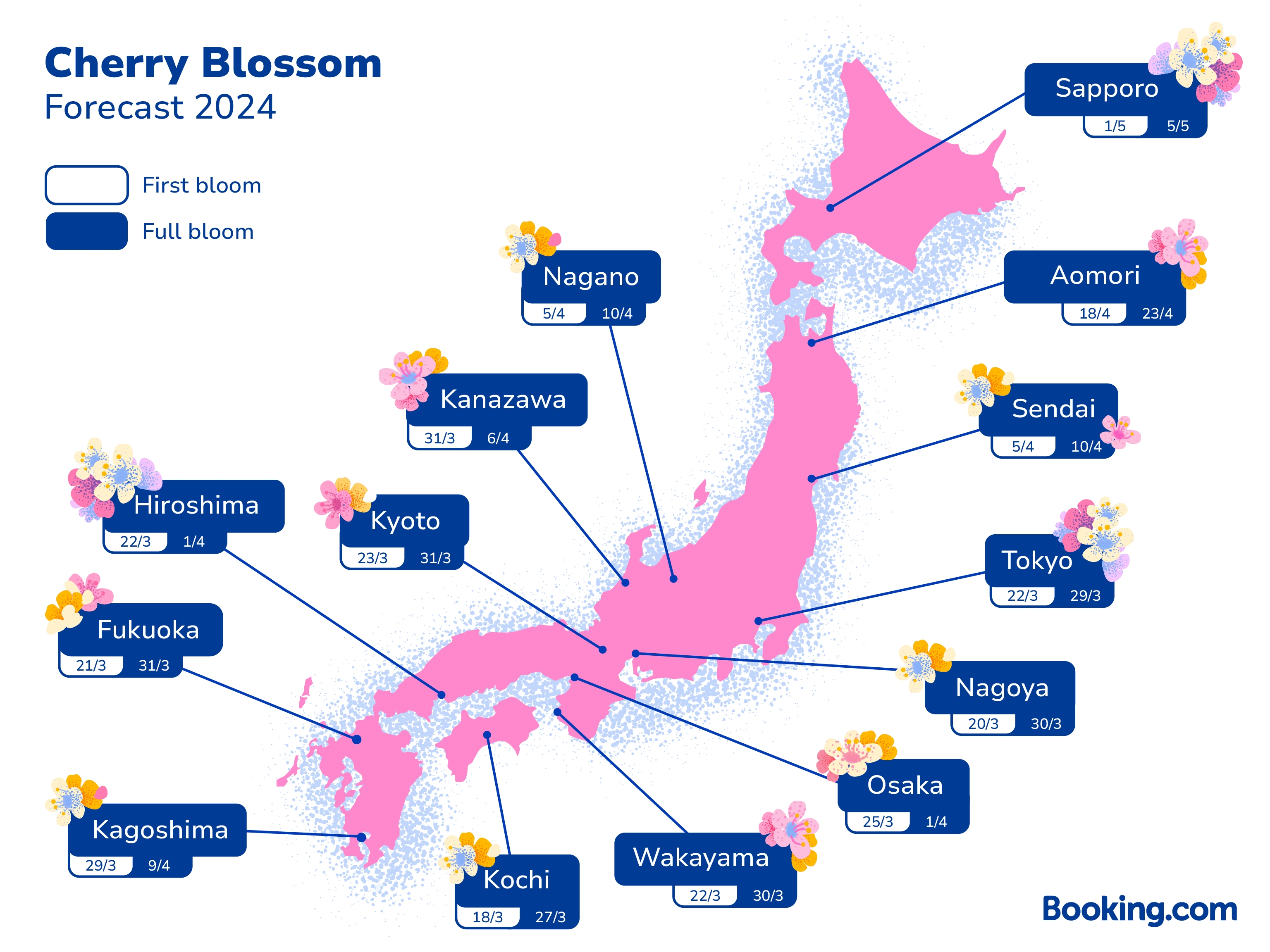This image showcases a detailed cherry blossom forecast for Japan in 2024. The map features the islands of Japan in a vibrant pink color, with light blue spots around them, and is labeled "Cherry Blossom Forecast 2024" at the top left corner. A legend on the map includes a white box labeled "First Bloom" and a dark blue box labeled "Full Bloom." The map is adorned with the names of various cities across Japan—Sapporo, Aomori, Sendai, Tokyo, Nagoya, Osaka, Wakayama, Kochi, Kagoshima, Fukuoka, Hiroshima, Kyoto, Kanazawa, and Nagano—each accompanied by their respective bloom dates. These city labels are set within dark blue boxes, featuring a small flower pattern in the corner, decorated with colors such as pink, orange, and hints of blue. Arrows point from each label to the respective city's location on the map. In the bottom right corner, "booking.com" is written in navy blue, indicating the source of the map and suggesting it helps travelers plan their visit to Japan for the cherry blossom season.